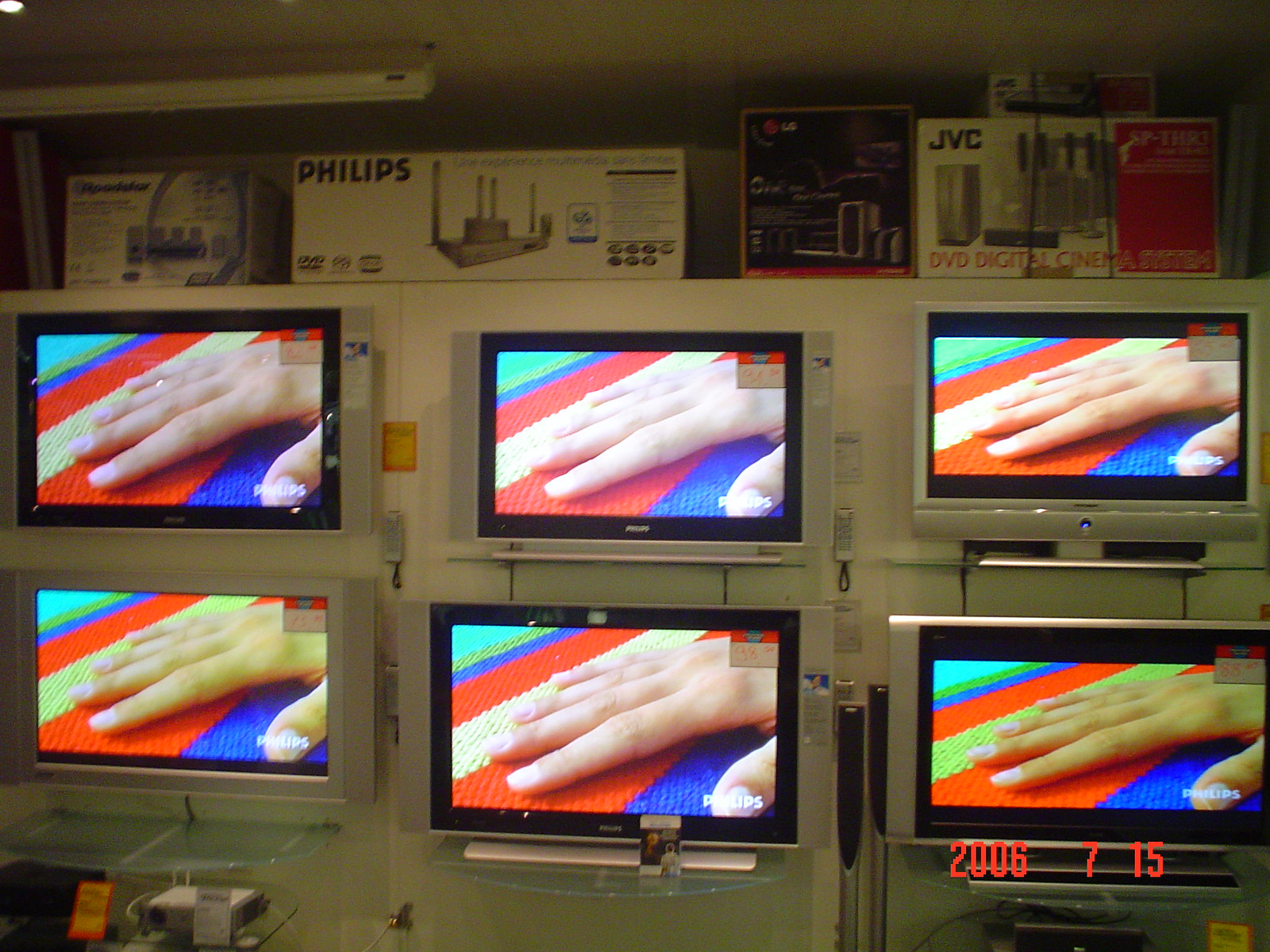The image, dated July 15, 2006, depicts six flat-screen televisions mounted against a white wall. Arranged in two rows of three, each television displays a slightly varied version of the same picture: a Caucasian hand against a multicolored background featuring red, yellow, green, and teal stripes. In the bottom right corner of each screen is a Philips logo. Below the televisions are glass shelves, and atop the wall behind them, various electronic device boxes from brands like Philips and JVC are visible. This setup resembles a display one might find in an electronics store or a warehouse, showcasing different television models and related products.